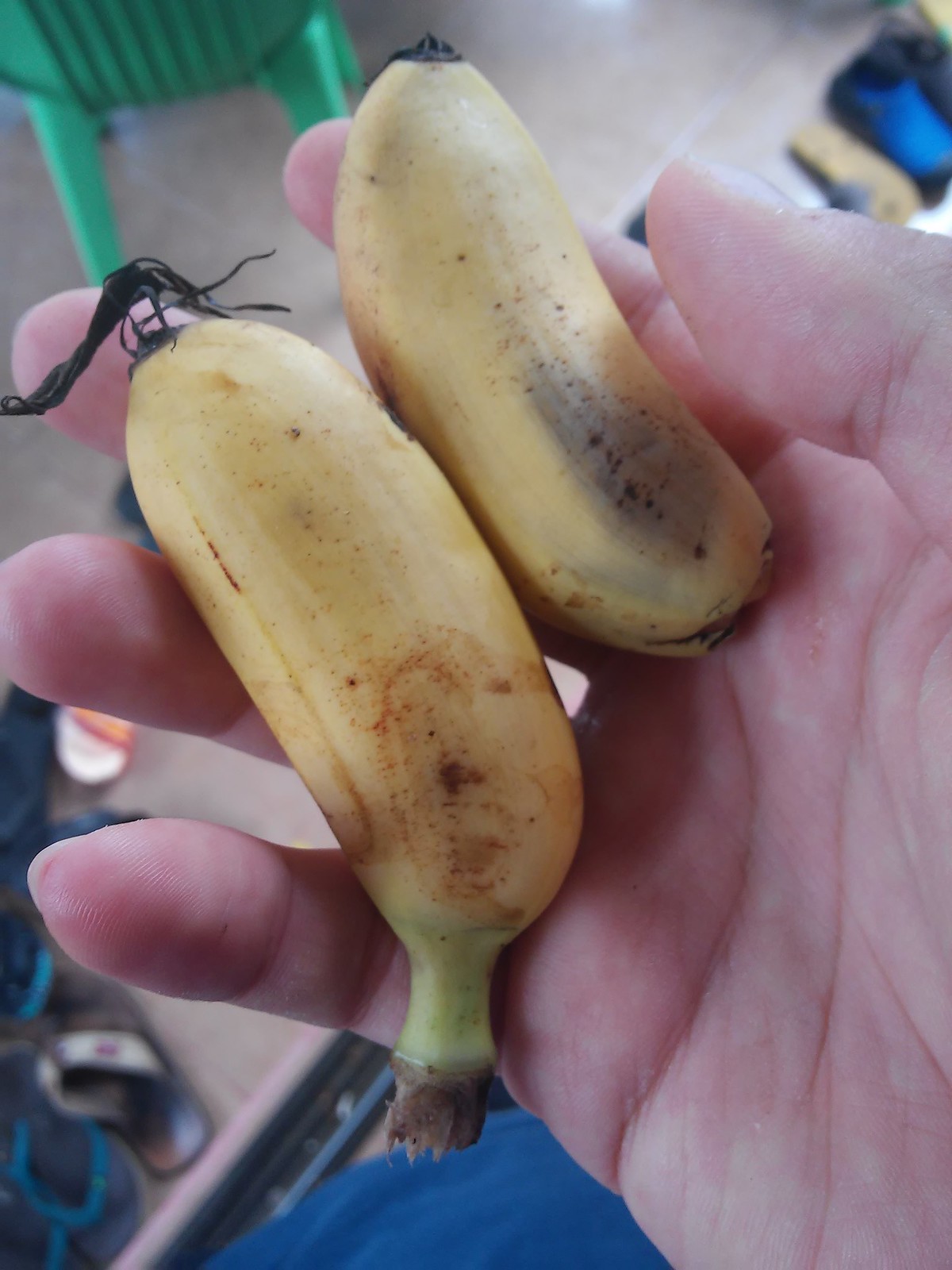This color photograph features a close-up of an individual's right hand holding two unusually shaped, small bananas in their kitchen. The focal point is the hand and bananas, which are prominently in the foreground. The bananas, both short and dumpy, differ from typical bananas. The one closest to the thumb has a noticeable bruise, while the second shows a green peeling end. Both exhibit yellow and black bruising, appearing overripe and unappealing. The surrounding kitchen is blurred, but visible details include a green plastic chair with three legs underneath the hand, and several flip-flops scattered on the floor—two blue, one white, one yellow, one black. The person's blue shirt slightly peeks into the frame, adding a touch of color contrast to the scene.